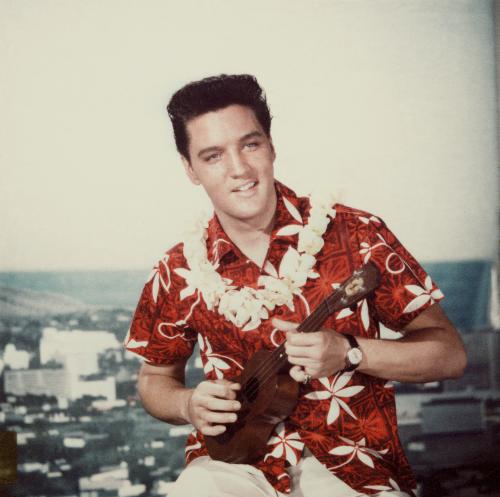In this vintage, square photograph from the 1950s or 1960s, a very young Elvis Presley is the main focus, seated and appearing to strum a small ukulele. He is clad in a short-sleeved red Hawaiian shirt adorned with white floral patterns, its open collar revealing a white lei draped around his shoulders. White trousers peek out from beneath his shirt, emphasizing his casual yet iconic look. Elvis's dark, styled hair and clean-shaven face are complemented by a black wristwatch with a white dial on his left wrist. His fingers are poised on the neck of the light brown ukulele, playing with his right hand. He is not looking directly into the camera; instead, his gaze is directed slightly to the side, his head tilted with a subtle, crooked smile that suggests he might be singing. The background features a cityscape, likely an illustrated backdrop with bluish-gray buildings and houses that transition into a white sky, giving the image a blend of realism and artistic backdrop. This setting, possibly in front of a window or an artificial scene, adds a nostalgic charm to the photo.